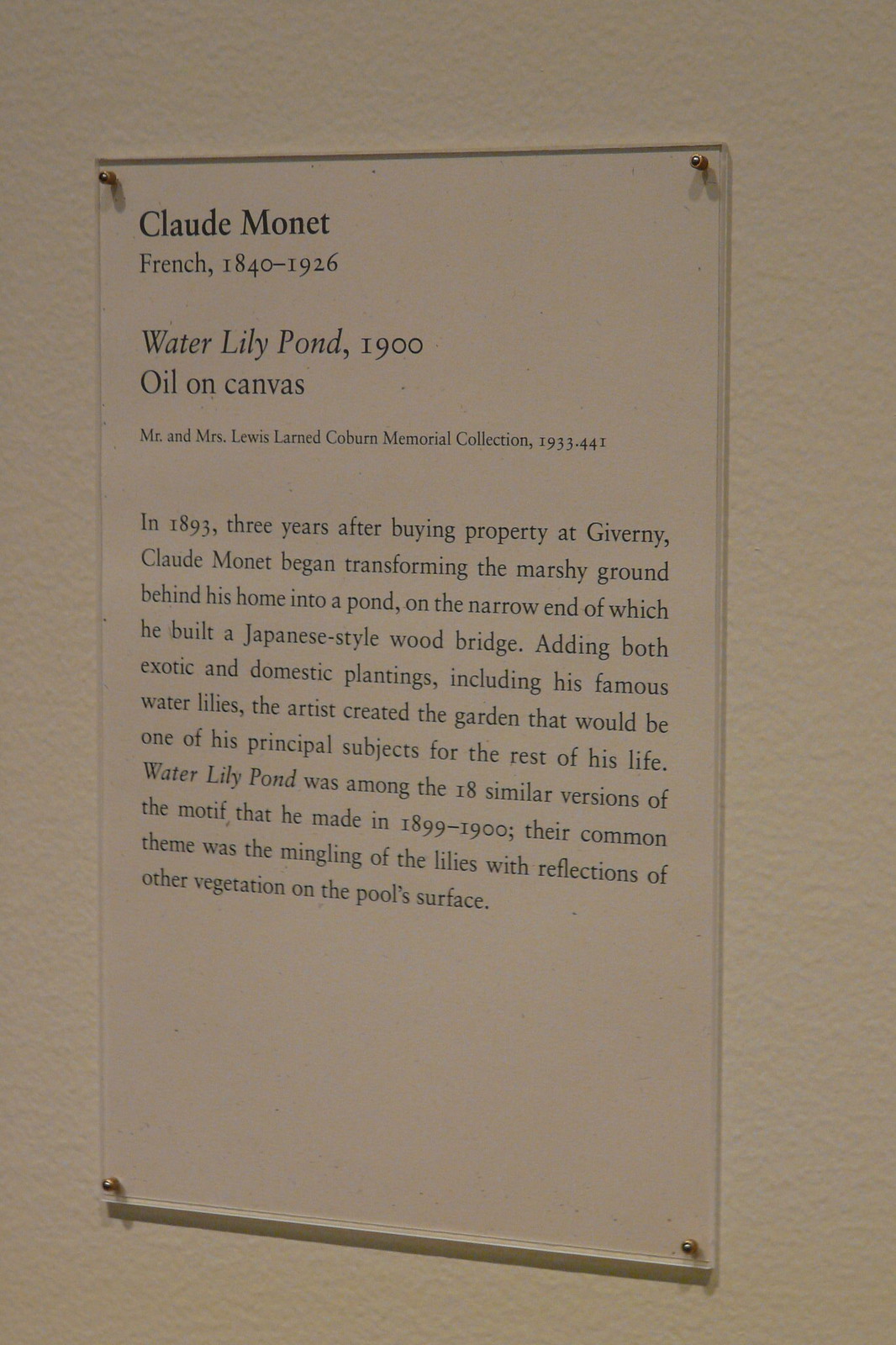This is an elegantly framed poster displayed on a light brown wall at an art gallery. Secured with four screws at its corners, it provides detailed information about a painting by Claude Monet. The heading, in bold black font, reads "Claude Monet" followed by "French, 1840-1926." Below, in italics, it identifies the artwork: "Water Lily Pond, 1900, oil on canvas." The poster notes that the painting is part of the "Mr. and Mrs. Lewis Learnéd Coburn Memorial Collection, 1933.44I."

A detailed biography in smaller print describes Monet's artistic journey. In 1893, three years after purchasing property at Giverny, Monet transformed the marshy ground behind his house into a pond, where he constructed a Japanese-style wooden bridge. He filled the pond with both exotic and domestic plantings, including his iconic water lilies. This garden became one of Monet's principal subjects for the rest of his life. "Water Lily Pond" was one of 18 versions of the motif created between 1899 and 1900, all featuring the mingling of water lilies with reflections of surrounding vegetation on the pond’s surface.